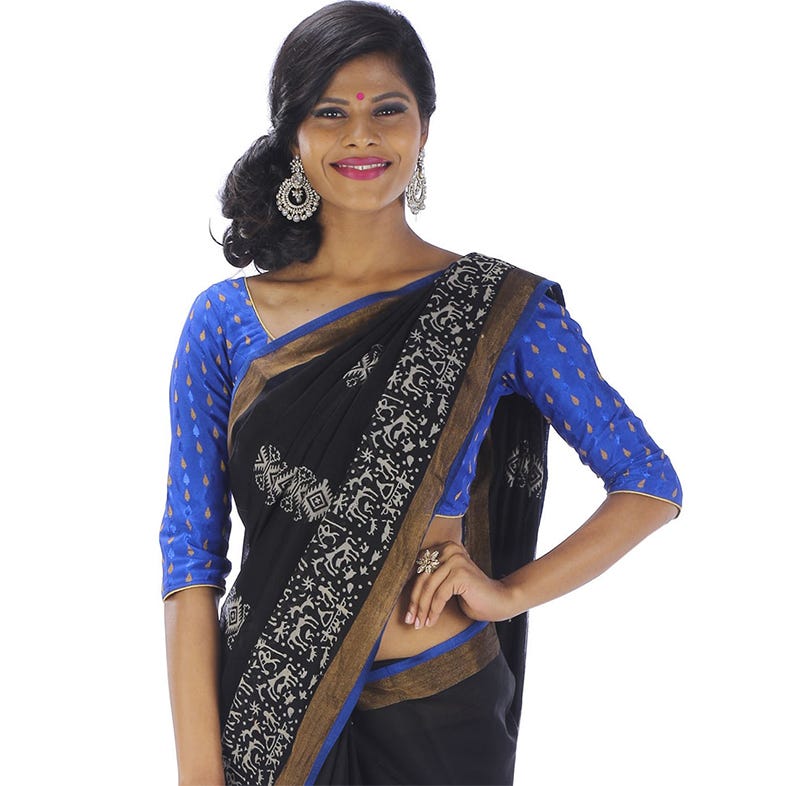This image features an Indian woman set against a plain white background, appearing as if cut and pasted into the scene. She is looking directly at the camera with a bright, cheerful smile, enhanced by her bright pink lipstick. Her long, thick black hair is elegantly tied back on the right side in a curly bun that grazes her shoulders. She is adorned with ornate, large silver hoop earrings, and a distinct red bindi marks the center of her forehead.

Her attire is an elegant blend of traditional and modern styles. She wears a three-quarter sleeve dark blue crop top with yellow diamond designs, which leaves her collarbones and part of her midriff exposed. Draped diagonally across her torso is a black sash with white designs, adding a sophisticated touch to her outfit. Below the sash, her black trousers are visible just above the waistline, partially covered by the garment. Additionally, she sports a ring on her left middle finger that features a floral design. Her overall look is completed with dramatic black eye makeup, complementing her polished and vibrant appearance. She stands confidently with her right arm down and her left hand resting on her hip.